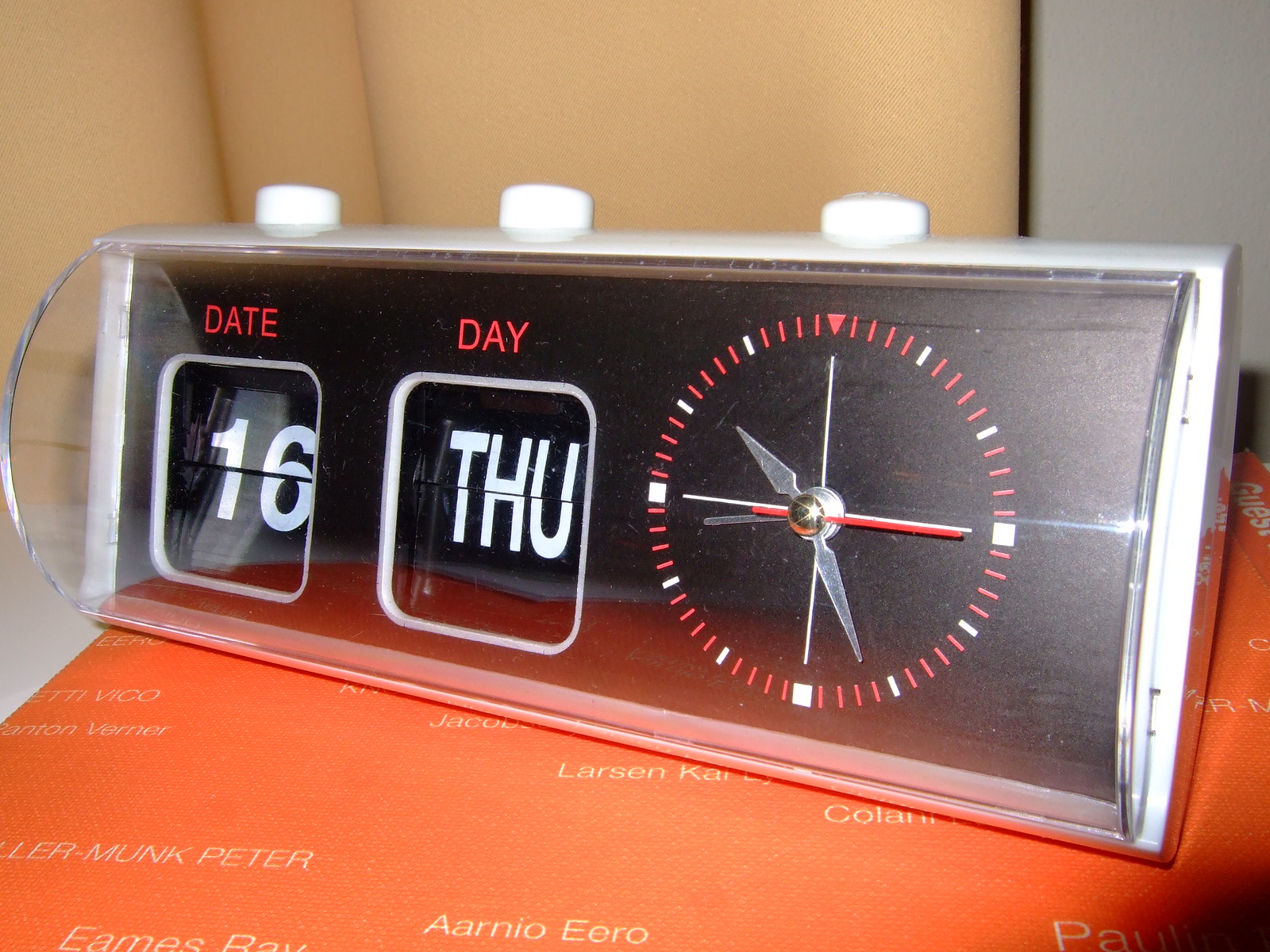The image is a close-up of a rectangular alarm clock resting on a piece of paper with an orangish-brown color. The paper lies at the bottom of the image and contains a series of names written in white text. Among these names, the only fully visible one reads "AARNIO EERO." 

The alarm clock has a silver-colored outer frame and a black background within its display area. The display is divided into sections: a square with the word "DATE" in red above it, showing the number "16," and another square next to it labeled "DAY," displaying the abbreviation "ATHU" for Thursday. To the right of these squares, there is a red and white wheel indicating the time.